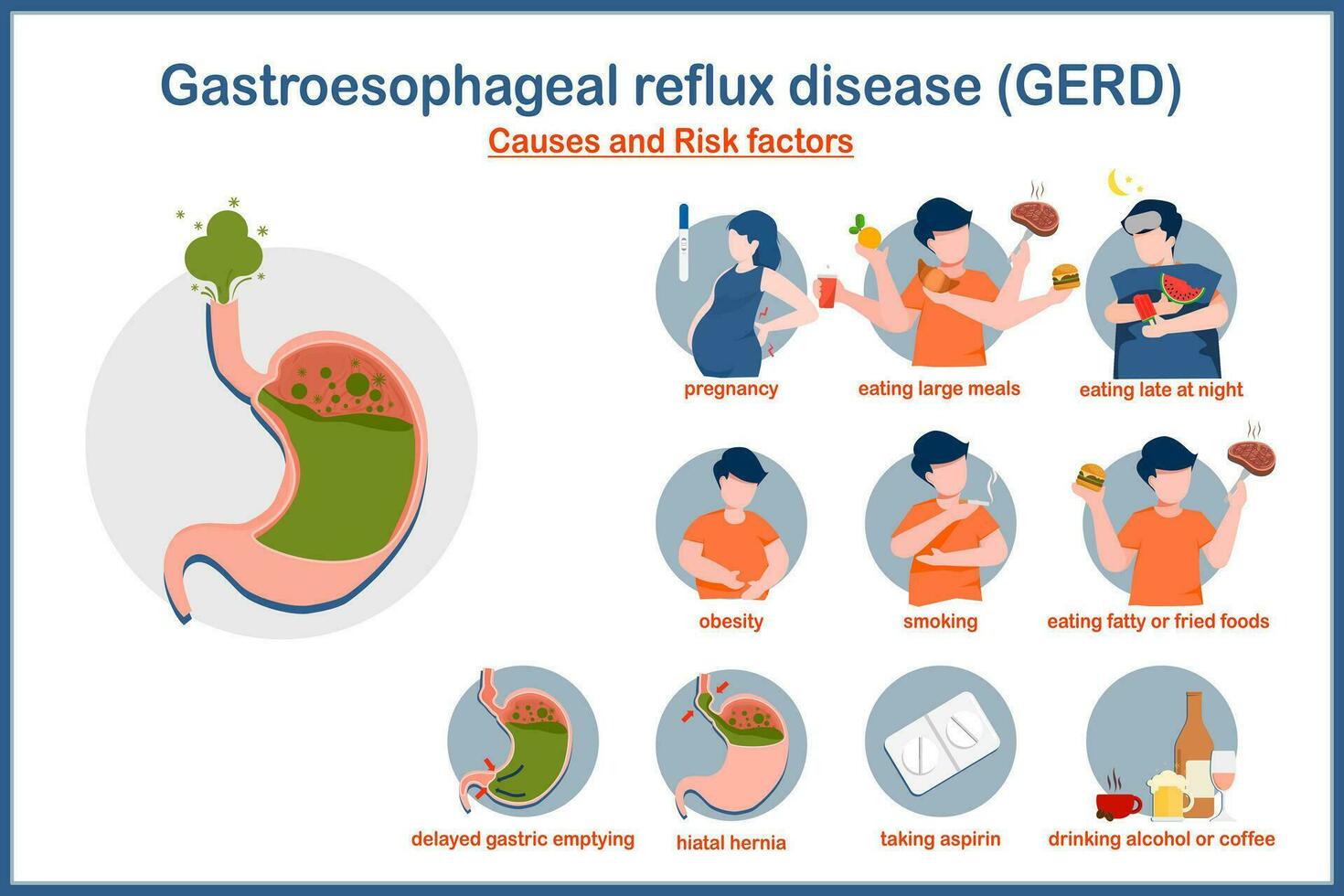The image is an educational poster about gastroesophageal reflux disease (GERD). It provides detailed information on the causes and risk factors associated with GERD, using fun and vibrant illustrations. The layout is distinctly colorful featuring predominant shades of green, orange, pink, blue, and gray. 

On the left side of the poster, set against a gray circular background, is a detailed illustration of a stomach. Inside the stomach, bright green stomach acid is depicted bubbling, with a broccoli-shaped cloud of acid rising where the esophagus would be. This visually represents the reflux action characteristic of GERD.

On the right side, each risk factor is illustrated with human figures placed against dark gray circular backgrounds. The first figure, a woman in blue, is labeled "Pregnancy." Next is a man with multiple arms, each holding different food items; he is colored in orange and labeled "Eating Large Meals." Below him is another man, lounging in bed under a blue blanket, labeled "Eating Late at Night." 

The second row of illustrations includes a man in orange labeled "Obesity," another man also in orange labeled "Smoking," and a man holding a burger and a steak labeled "Eating Fatty or Fried Foods."

The bottom row features the stomach again against a gray background with the label "Delayed Gastric Emptying," an illustration of a stomach labeled "Hiatal Hernia," two tablets against a background labeled "Taking Aspirin," and finally, a bottle and glasses labeled "Drinking Alcohol or Coffee."

The entire poster is prominently outlined in blue with dark blue ink highlighting the title at the top. This vibrant and detailed visual guide effectively communicates the various activities and conditions that can lead to GERD.